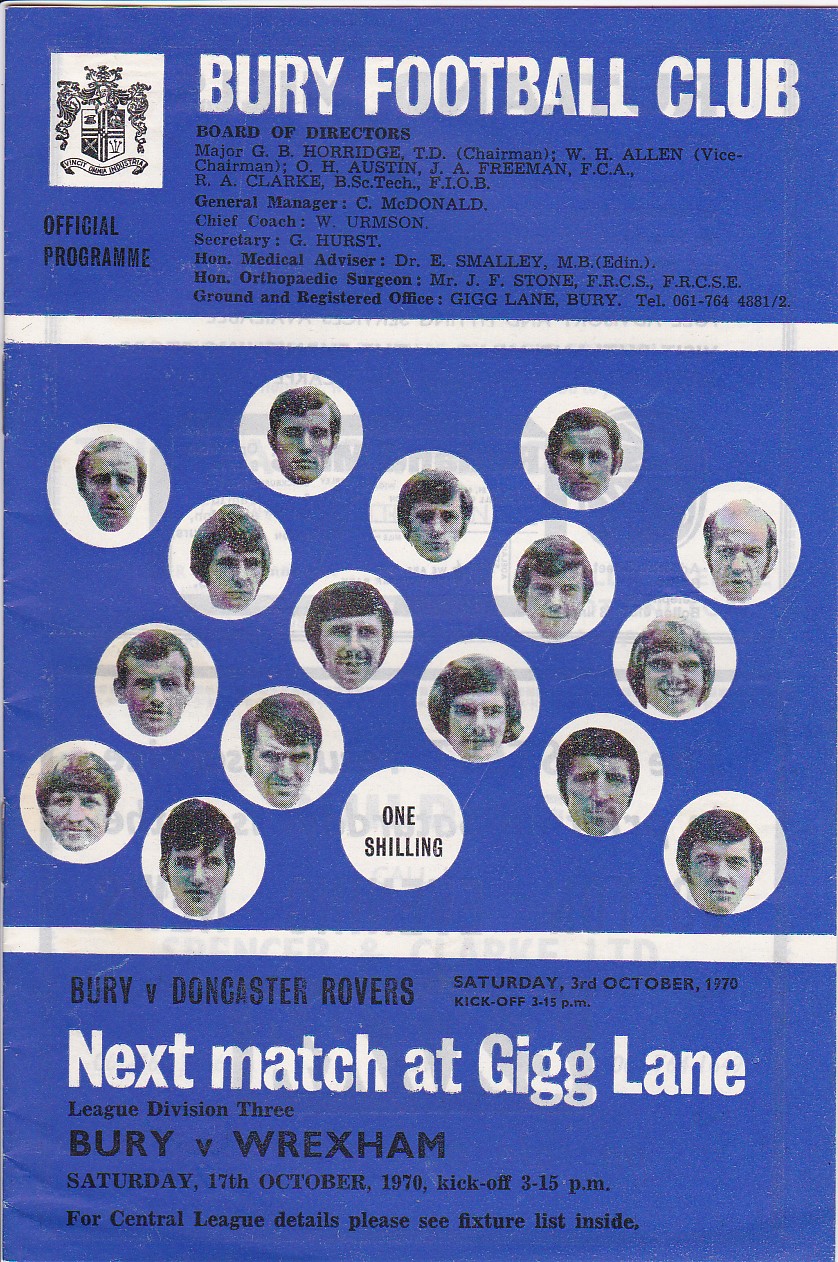The cover of the official program for Burry Football Club features a deep blue background. At the top left, there is the Burry Football Club's logo, depicted as a white crest with a black sketch in its interior. Adjacent to the logo, boldly stated in white lettering, is "Burry Football Club." Below the club's name, in smaller black text, it reads "Board of Directors." Directly beneath the logo, it proclaims "Official Program" in black text. 

Following this, a horizontal white bar separates the titles from the main content. Centered on the page are black and white photographs of the players’ faces, each encased in white circles set against the blue background. There are approximately 15-16 player images displayed. In the midst of these players' images and enclosed within a white circle, the cost "One Shilling" is indicated in black text.

Towards the bottom, another white bar appears, below which bold white text announces, "Next Match at Gig Lane." Further below, in smaller black text, the details of the upcoming game are provided: "Burry vs. Wrexham, Saturday, 17th October 1974, kickoff 3.15pm. For central lesion details please see fixture extension inside."